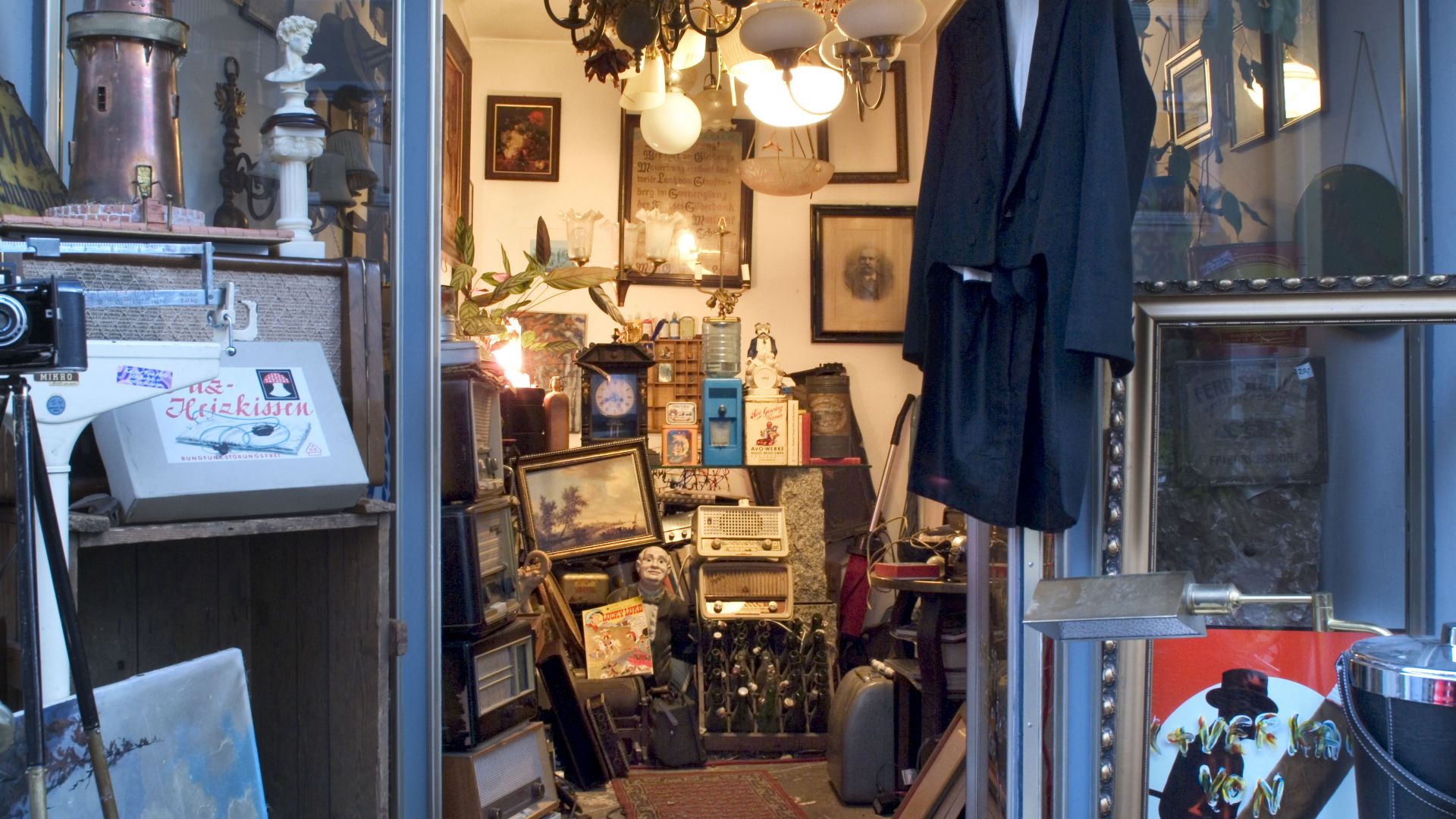This image captures the cluttered interior of a small antique shop or storage room, brimming with a plethora of vintage items and knickknacks. The scene is dominated by various ceiling fixtures and chandeliers, some illuminated, creating a nostalgic ambiance. On the left side, shelves are stacked with an assortment of items including a blue vintage water dispenser, a copper lighthouse figurine, and a statue resembling a Roman figure. Among the clutter, there is a gray box with a mushroom logo, and several radios huddled together, along with a collection of wine glasses. 

The room is further adorned with numerous picture frames showcasing both old black-and-white photographs and paintings, along with a few framed portraits. On the right, there stands a glass display case and a red vacuum cleaner with a metal rod. The wall's white surface provides a contrast to the dark, antique wooden frames of the clocks and pictures, including one with a depiction of trees. Additionally, a black robe hangs from the ceiling near a poster. The overall scene presents a treasure trove of storied objects, evoking a sense of curiosity and historical intrigue.